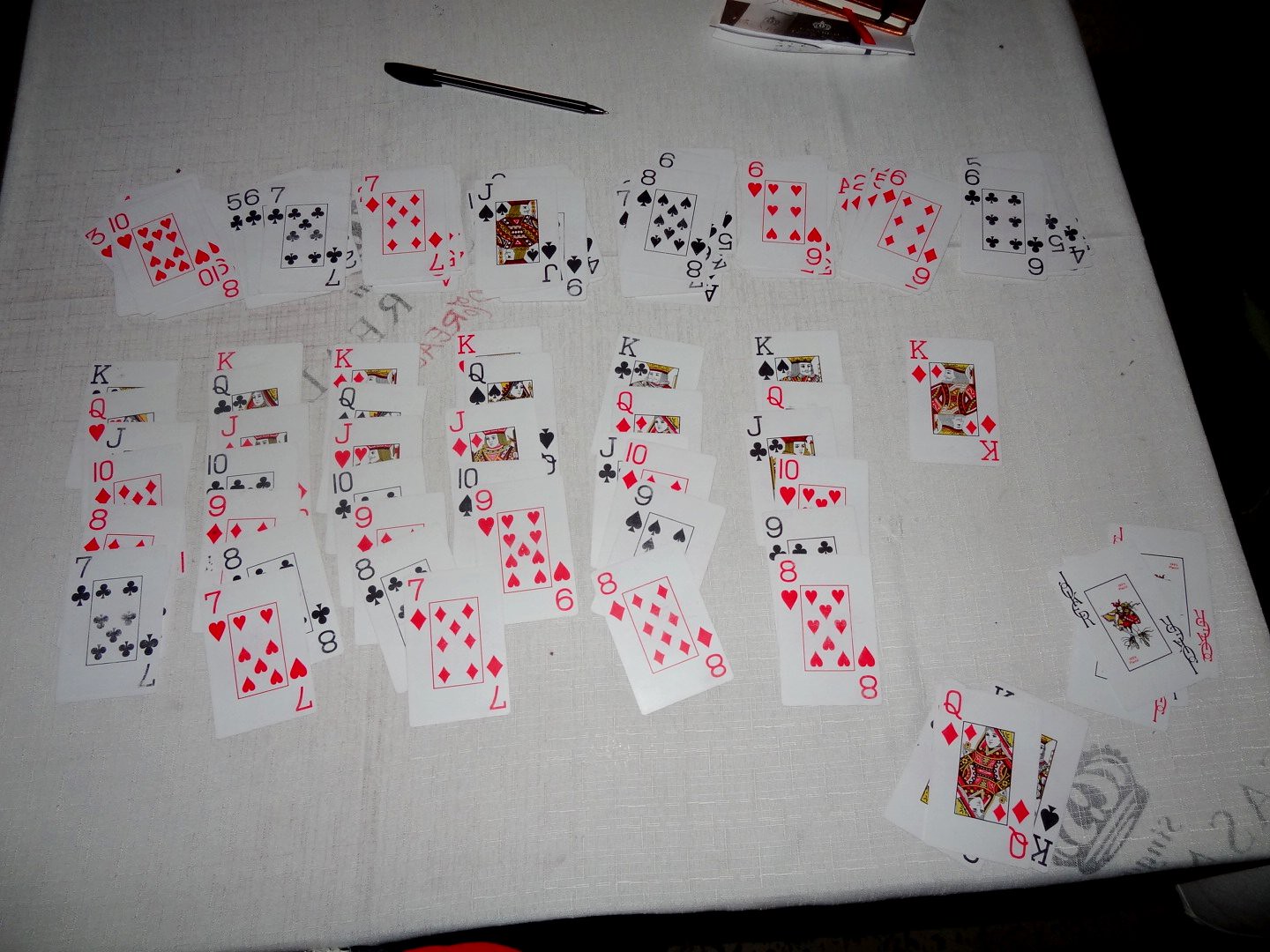A photograph features a white canvas board positioned in the middle of a dark black or brown floor. Across the board, playing cards are meticulously arranged in a traditional solitaire layout, with seven stacks laid out horizontally. The cards, appearing to be from a double deck, display a variety of suits and ranks, including multiple kings of different colors and shapes, as well as numerous spades, clubs, and diamonds. The suits are grouped at the top in a striking pattern: red, black, red, black, black, red, red, and black. A black pen is placed diagonally across the board. Toward the bottom of the board, several kings are stacked together, accentuating a crown-like print alongside some writing, adding an artistic element to the image.